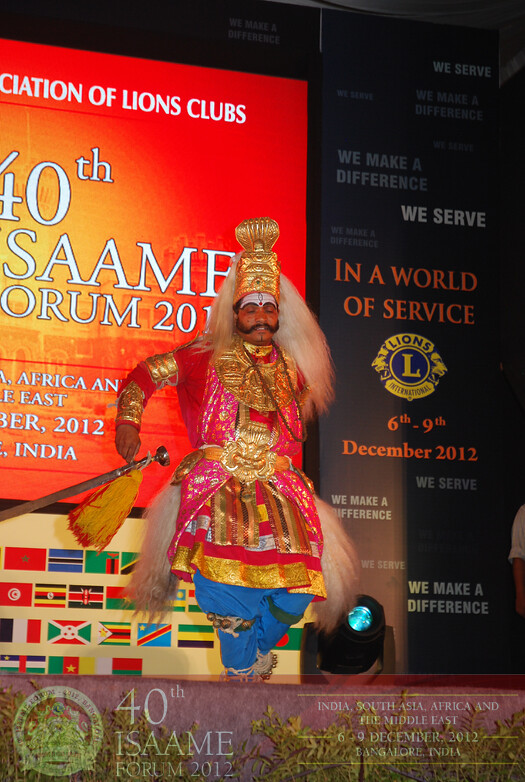The image captures a man on stage, seemingly dancing in traditional Indian attire at the 40th ISAM Forum held from December 6-9, 2012, in Bangalore, India. The man is adorned in a vibrant costume that consists of a long red and gold shirt-dress embellished with intricate gold details, and blue baggy pants. His elaborate outfit also features elements of pink, yellow, and white fur accents. He wears an eye-catching gold headdress reminiscent of a traditional helmet, from which wispy hair-like decorations flow. His face is distinguished by a long handlebar mustache extending to his sideburns. In one hand, he holds what appears to be a golden walking stick or sword, adding to his regalia. The stage is lit by a spotlight and adorned with numerous banners and signs. The text on the left of the image solidifies the event’s context, reading: "40th ISAM Forum 2012, India, South Asia, Africa, and the Middle East, 6-9 December 2012, Bangalore, India," while additional signage includes the slogan "We make a difference, we serve in a world of service, Lions International." The detailed background and the man's ornate attire suggest he is performing a traditional dance, making the scene both culturally rich and visually captivating.